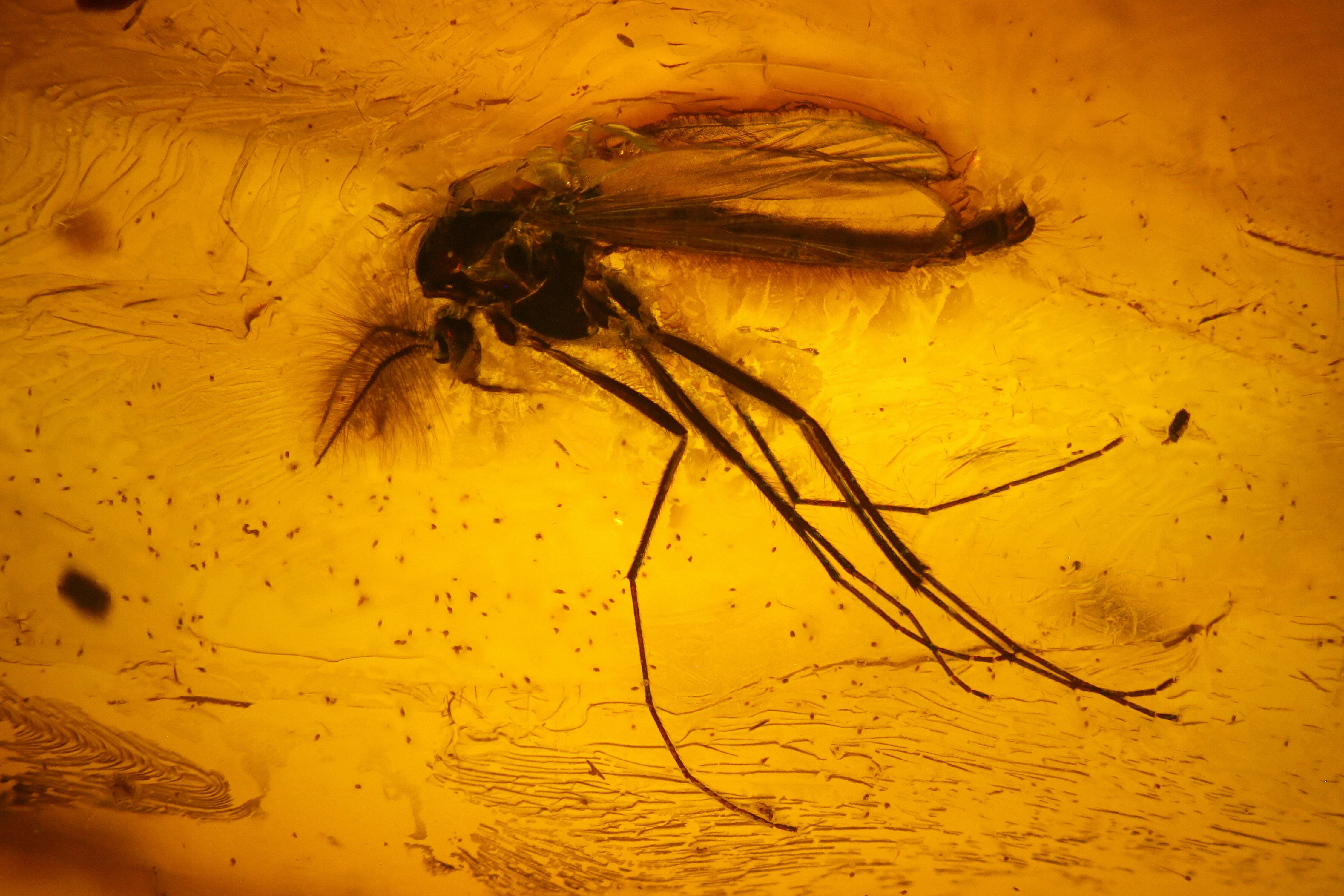A detailed, close-up photograph depicts an insect, likely a mosquito, preserved in amber. The insect's body is suspended within the yellowish-gold, glassy, and crystalline texture of the amber, which shows wavy sections and scattered dark brown specks. The insect features long, jointed legs, estimated to be around 3 inches in length, and transparent wings that span several inches, emanating from its back. Its body is primarily a golden color, with part of it appearing darkened. Visible near the head section are what appear to be hairy antennae. The overall scene is enveloped by the amber, giving the background a consistently golden hue with various textures and particles trapped within.